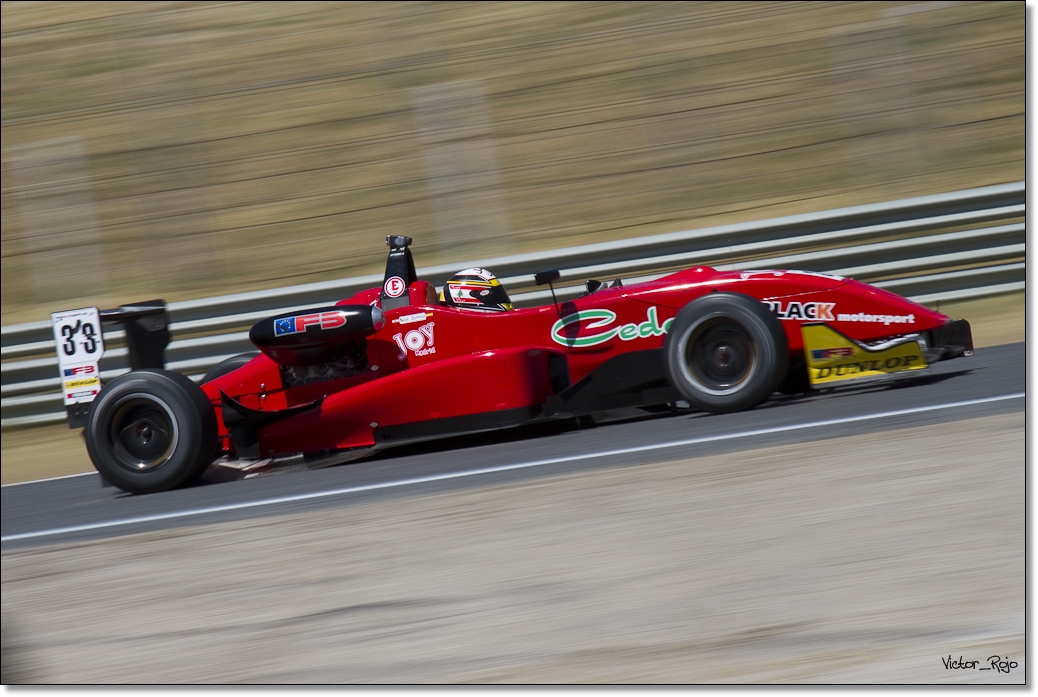This wide rectangular image captures a Formula One race car speeding down a narrow gray road marked with white paint. The car, a vibrant red, is equipped with various sponsor logos, including partially legible ones like Joy, something black, and possibly Seed. A prominent black wing, bearing the designation "F5", extends from the car. The driver, whose top helmet design includes white, yellow, black, red, and a bit of blue, is tightly strapped into the cockpit with the visor down. A GoPro camera is mounted on the roll bar, facing forward, and a rear view mirror is visible on the side. The car, extremely close to the ground with black wheels, blurs past the metal fence composed of three horizontal barriers, against a background of blurry yellow and green hues, adding to the sense of high speed. A blurry sign that reads "3S" flashes by, while a yellow "Dunlop" and green "CEDO" label are also spotted on the car. The image is credited to Vitor Rojo, whose name appears subtly in the very right-hand corner.